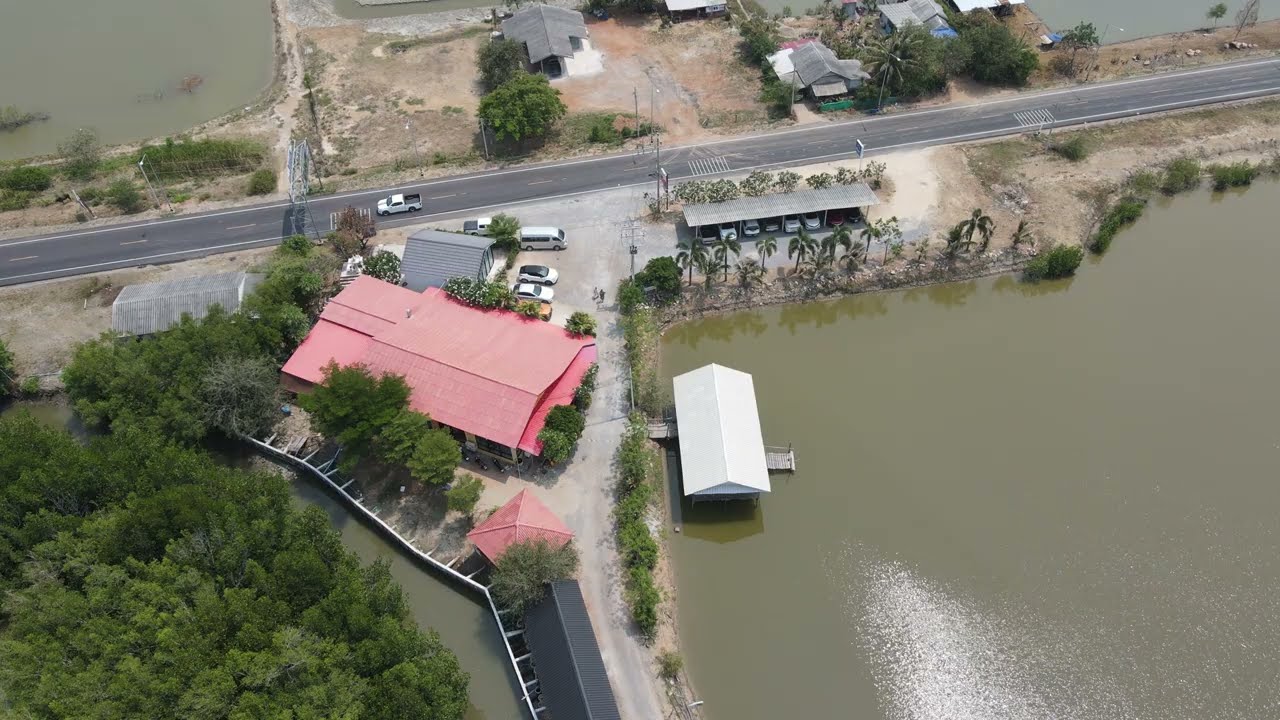The aerial photograph captures a business-like building with a striking red roof, positioned centrally near a prominent body of water located mainly in the bottom right corner. Surrounding the building, which is accompanied by a few parked vehicles, are various other smaller buildings mostly found towards the top part of the image across an unpaved area. A single-lane road cuts horizontally across the top of the image, where a truck is seen driving. The scene is enhanced by the presence of lush palm trees at the edges and a dense cluster of trees in the lower left, adding a touch of greenery to the otherwise seemingly desert-like terrain. The setting is outdoors, under the clear daylight, showcasing the hues of green, gray, white, red, yellow, and tan, indicative of a quiet, perhaps semi-rural area. The water extends subtly to other corners of the image, suggesting a picturesque, delta-like environment.